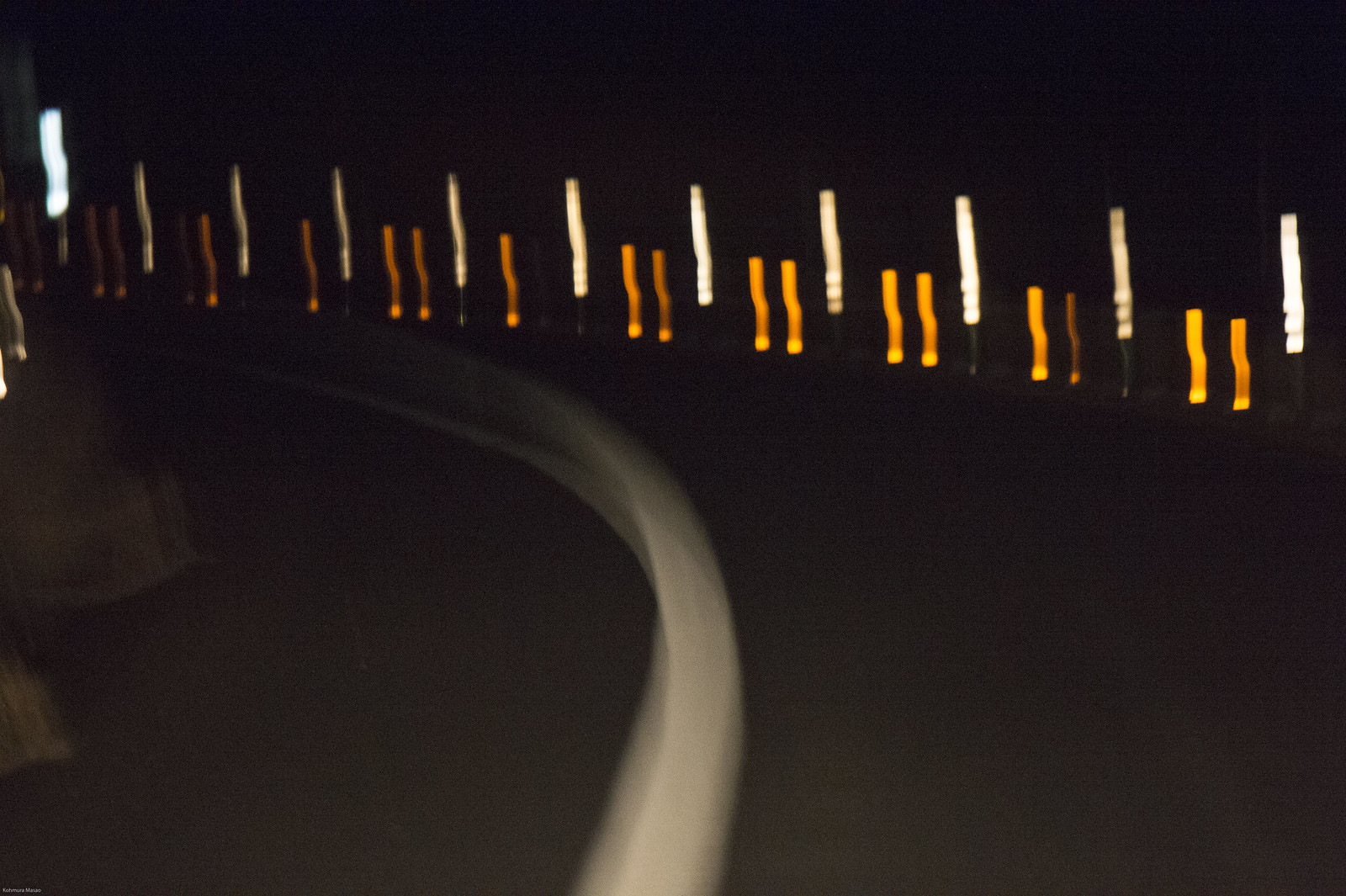This night-time photograph has a predominantly black background, capturing a mysterious and somewhat abstract scene. A defining feature, which could be a concrete wall or possibly a rubber strip, arches from the lower center of the frame and curves toward the upper left side. This structure obscures a portion of what appears to be a roadway. Adding to the complexity of the image, the upper section features a series of alternating lights. These lights, composed of white and orange stripes, stretch from the upper left corner toward the middle right. The orange lines intriguingly bend around an unseen barrier, altering their angle at the center of the photograph. The interplay of light and shadow creates an enigmatic and visually arresting composition.